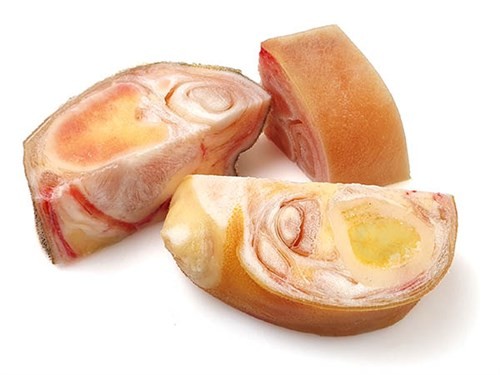This image features three half-moon-shaped slices of an undisclosed fruit or meat, artfully arranged on a white surface. The outer layer resembles an orange peel, implying a citrus characteristic. The interior is detailed with multi-layered cross-sections comprising an orange-hued outer part, a white middle layer, and a peachy to yellowish orange core. One slice stands upright, adding visual interest, while the other two lie flat, showcasing the range of internal textures and colors, suggesting an intricate structure possibly indicating "fruits within a fruit" or intricate muscle fibers. The precise nature of these layers and their taste differences remain unknown, but the arrangement and vivid color palette create a visually intriguing composition.